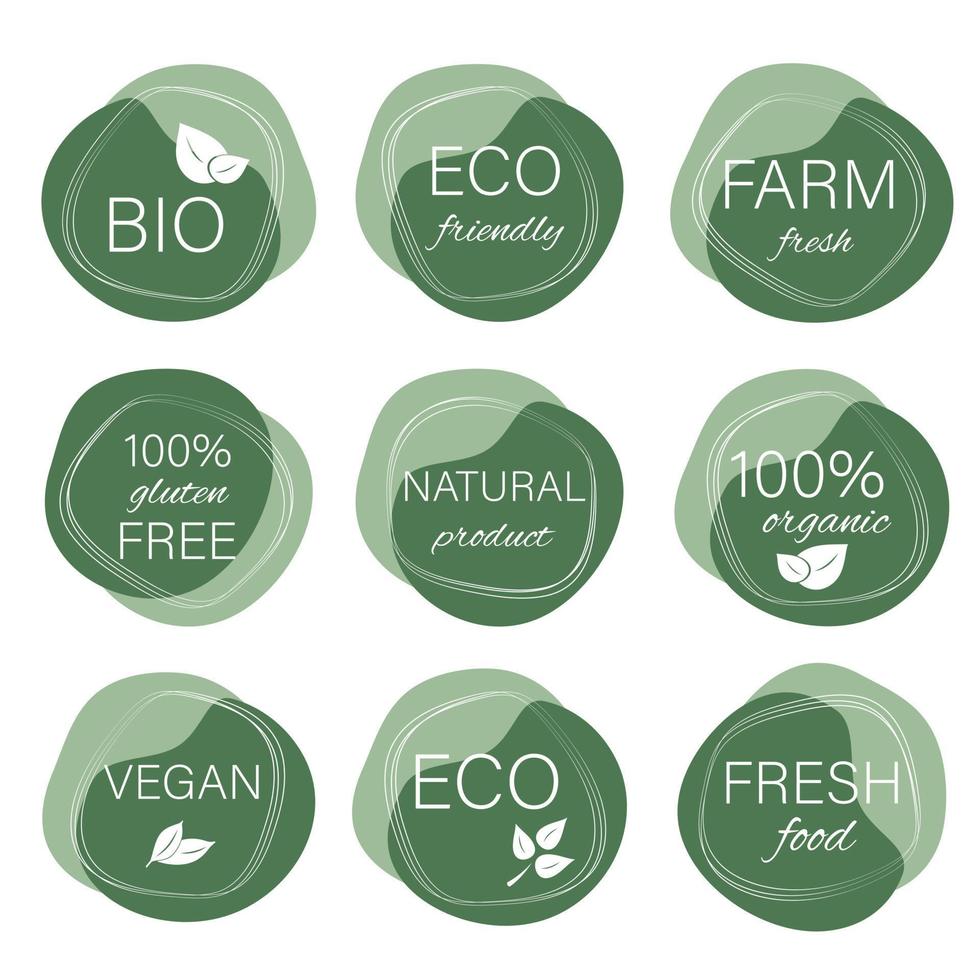This image features a 3x3 grid of nine green circles, each adorned with white text that highlights various eco-friendly and health-oriented attributes. Starting from the top left and moving right, the circles are labeled: "Bio," "Eco-friendly," and "Farm Fresh." In the middle row, they are: "100% Gluten-Free," "Natural Product," and "100% Organic" (accompanied by a small leaf graphic). The bottom row includes: "Vegan," "Eco" (with a three-leaf icon), and "Fresh Food." The circles are uniform in shape, a blend of dark and light green, and the consistent use of white text and occasional leaf imagery suggests a promotion of sustainable and healthy food products.